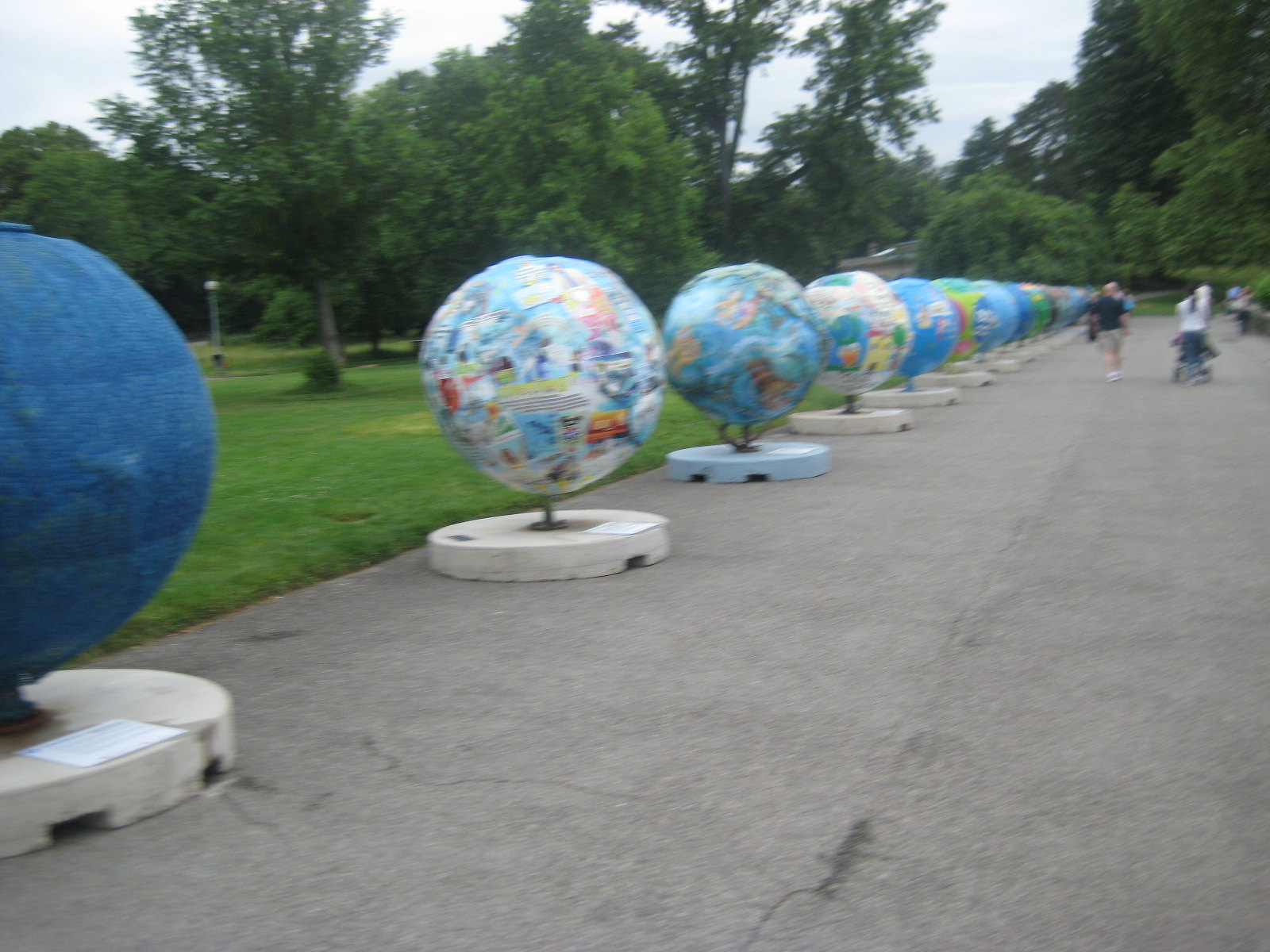The color photograph portrays a slightly blurry scene captured in a park setting. Dominating the right half of the image is a broad, gray asphalt path, reminiscent of a wide pedestrian lane. On this path, at least 15 globe-shaped statues are lined up in a row. These spheres, each perched on a round pedestal, vary in design and artistic interpretation. The globes are adorned with various patterns: the one on the far left, partially visible due to cropping, appears solid dark blue, while others are decorated with vibrant blues, whites, and greens through techniques that suggest painting or decoupage. Some globes display a smooth surface, while others have textures that might depict continents or other forms of artistic treatment.

To the left of this row of globes, a grassy lawn leads up to mature green trees, enhancing the park-like ambiance. In the backdrop, you can spot a low building with a skylight, possibly a public restroom. Toward the upper right side, distant pedestrians, including a woman pushing a baby carriage, walk along the asphalt path, offering a sense of scale. These enormous globe statues, estimated to be five or six feet tall, exhibit diverse and imaginative designs, indicating contributions from different artists or groups.